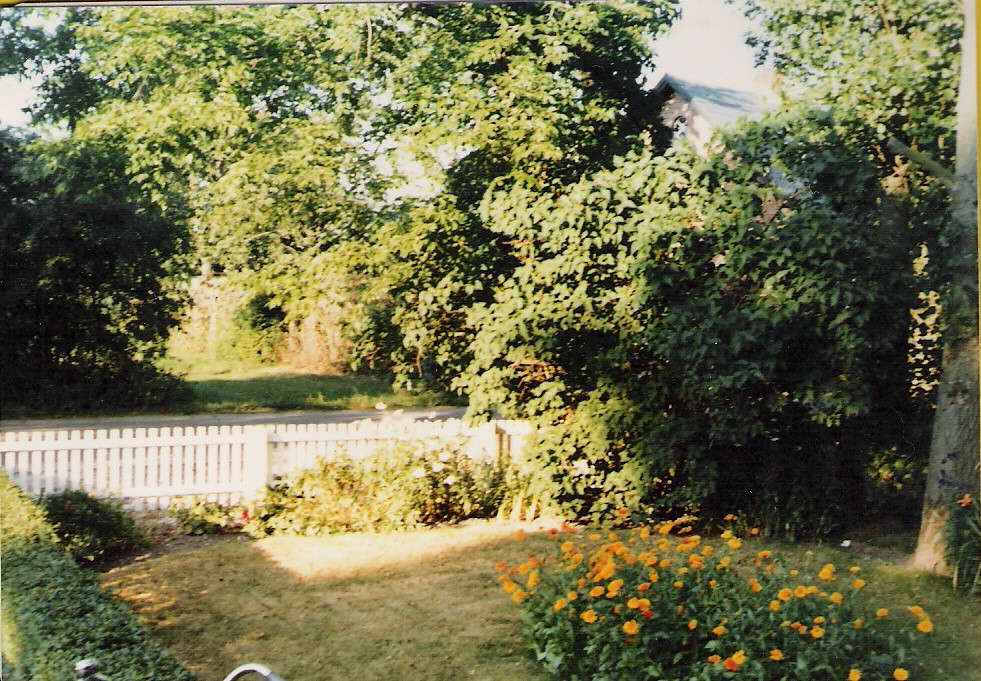This photograph, taken on a bright and very sunny day, depicts a serene yard or garden scene. The lush, green trees and large bushes indicate it's spring or summer, with the cloudless, vivid blue sky adding to the vibrant atmosphere. In the foreground, there is a neatly white picket fence that extends from the left side of the image to about two-thirds of the way across. The waist-high fence is partly obscured by well-maintained shrubs and greenery. Along the left side of the fence, a tidy row of shrubs leads up to a grassy area in the center, which is bathed in sunlight. Close to the middle right, a cluster of orange flowers stands out vividly among more shrubbery, while towards the front bottom of the photograph, a patch of yellow flowers with green petals catches the eye. Beyond the white picket fence, a small portion of a paved road is visible, with a grassy field and additional vegetation extending further back. In the upper right corner, partially hidden by the dense foliage, the roof of another house is evident.